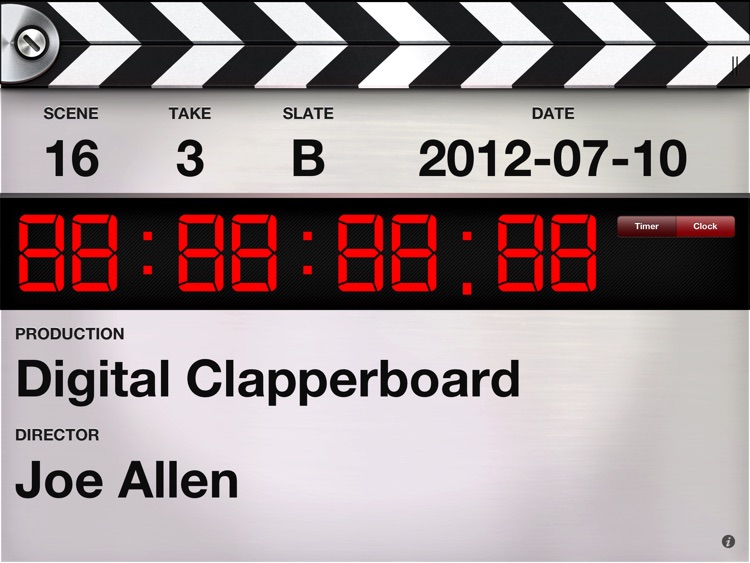The image depicts a digital recreation of a clapperboard used in film or video production. The top half features the traditional black and white striped clapper area that opens and closes, used by directors when they say "action." Below this section, on a silver background, it reads: Scene 16, Take 3, Slate B, dated July 10, 2012. Additionally, there's a digital clock below displaying the default time "88:88:88," capable of being set to either clock or timer mode. On the bottom half of the clapperboard, in black text, the production credits are listed: "Production: Digital Clapperboard, Director: Joe Allen." In the bottom right corner, a small clickable icon likely offers more information or context in an interactive format. The clapperboard serves as a placeholder reference for the editing team, indicating the start of a project.